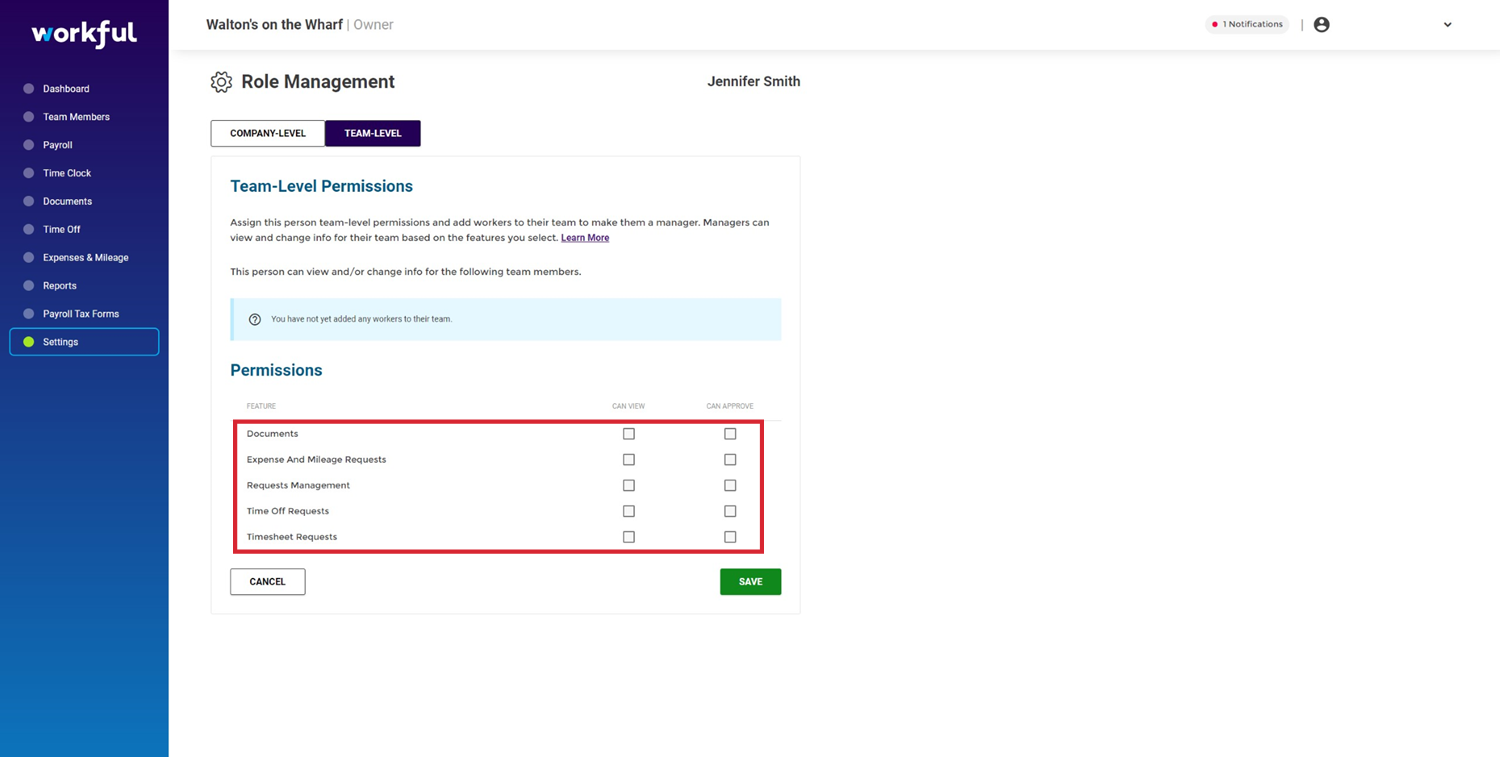The screenshot showcases the interface of a software named WORKFUL, designed for work and project management. On the far left of the screen, a vertical banner spans from top to bottom, displaying a gradient that transitions from dark blue at the top to light blue at the bottom. The name "WORKFUL" is prominently displayed in small caps white letters, except for one half of the "W" which is colored in the same light blue as the bottom of the banner, suggesting stylistic branding. 

Below the banner, a menu provides various options: Dashboard, Team Members, Payroll, Time Check, Documents, Time Off, Expenses, followed by an unreadable small text option, and concluding with Reports, Tax Forms, and Settings. 

A section details information about the ownership and management roles, stating that Walton's on the Wharf is the owner and Jennifer Smith handles role management. A portion labeled "TEAM LEVEL" and "TEAM LEVEL PERMISSIONS" discusses permission settings, with small text elaborating on the specifics. 

Permissions can be individually set for categories such as Documents, Expenses, Mileage Requests, Management Requests, Time Off Requests, and Timesheet Requests. A red text box highlights some of these permissions, indicating they are modifiable. At the bottom of the settings panel, there are options to either cancel or save the adjustments made.